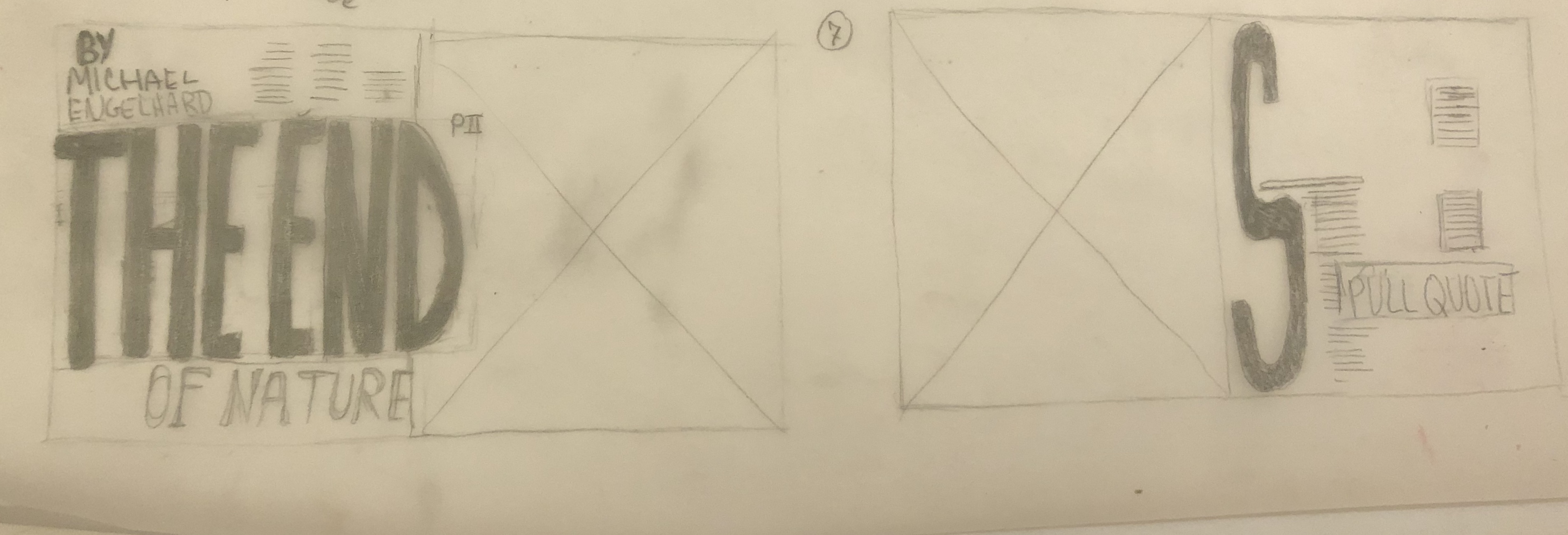In this image, we see a photograph of a hand-drawn sketch on a piece of paper, likely outlining the initial planning stages of a comic book. The drawings appear to be done in pencil, featuring two large rectangles that are each divided in half. 

In the left rectangle, the right-hand square is marked with a large X. To the left of this rectangle, the words "By Michael N. Gillard" are legibly written, suggesting the author's name. At the bottom left corner of this sheet, the phrase "The End" is prominently displayed in bold script, followed by the same phrase in a smaller text, likely denoting completion or finality in the comic's narrative. Additionally, there is a letter "P" accompanied by an unspecified symbol.

The right rectangle showcases the number "7" encircled at the top, hinting that this might represent the seventh page or panel of the comic. Within this rectangle, the left square is also X'd off, while the right square contains a large letter "S" and a box with the text "Pull Quote" within it. Scattered across the page are various lines, some shaded in, which likely indicate areas where text or artwork will be inserted in the future.